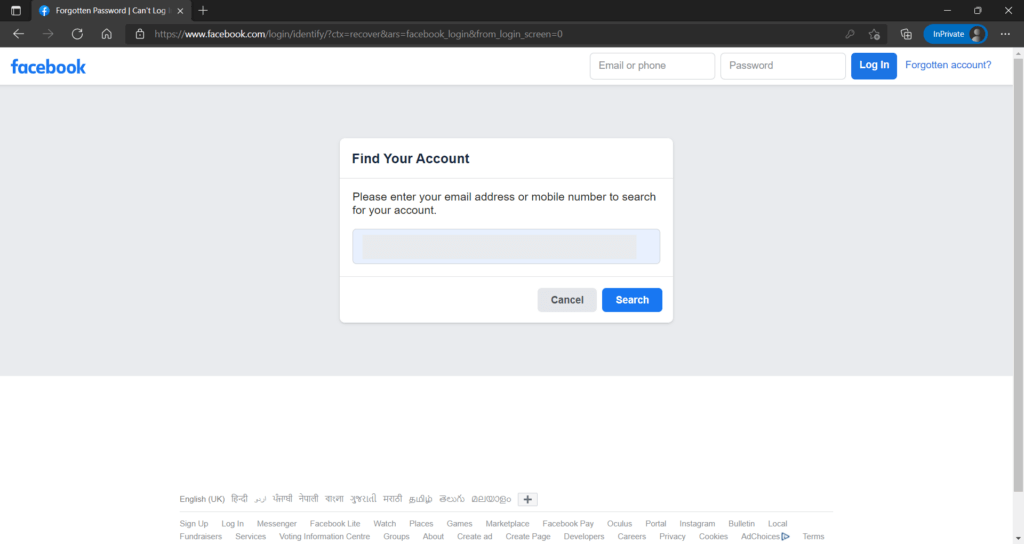The image is a screenshot of a Facebook page displayed in a web browser with a black background. At the top, characteristic icons include a home icon and a padlock next to the address bar, which contains "Facebook.com." On the far right side, a blue tab labeled "InPrivate" features a circle with a generic person icon inside it. Below, a white border spans the page.

In the top left corner, "Facebook" is written in blue text. On the right side, two text boxes are present: one labeled "Email or Phone" and another labeled "Password," accompanied by a "Log In" button and a "Forgotten account?" link.

Central to the page, against a gray backdrop, is a prominent white rectangle. At the top left of this rectangle, bold text reads "Find Your Account." Below, the instructions request: "Please enter your email address or mobile number to search for your account." A gray search box with no text entered sits underneath this.

To the right of the search box, two buttons are aligned horizontally. The first button, in gray, reads "Cancel," while the adjacent blue button reads "Search."

At the very bottom of the page, small text denotes "English (UK)" followed by several foreign languages. Links for various Facebook services, such as "Sign Up," "Messenger," "Watch," "Places," and "Portal," are listed in small text.